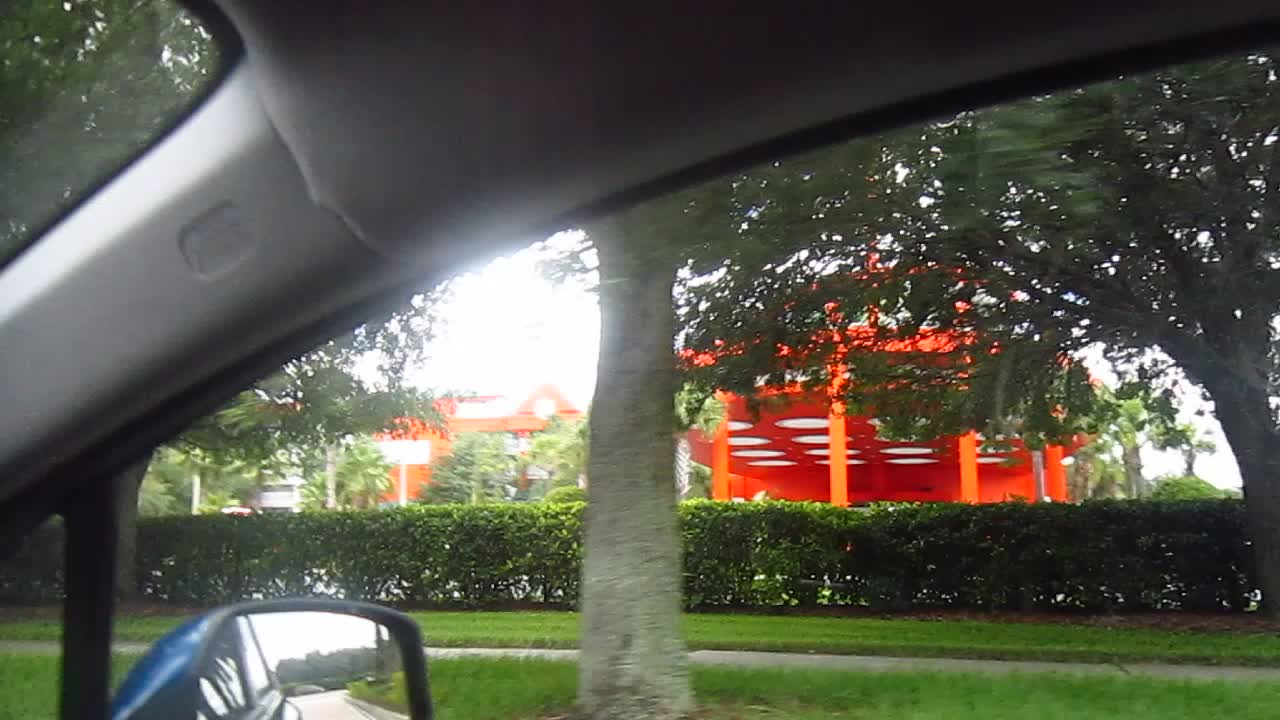This photograph, taken from inside a car, captures the reflection of the vehicle's window and interior elements, including the car's roof and the rearview mirror visible at the side. The scene outside the car appears to be a street-side view, where the vehicle is parked. Surrounding the car is a landscape featuring lush grass, a few scattered trees, and a row of bushes that line the foreground. A sidewalk separates the greenery from a prominent orange structure in the background. This orange structure appears to be a building, augmented by an additional elevated orange feature supported by pillars, contributing to a whimsical, playground-like appearance.